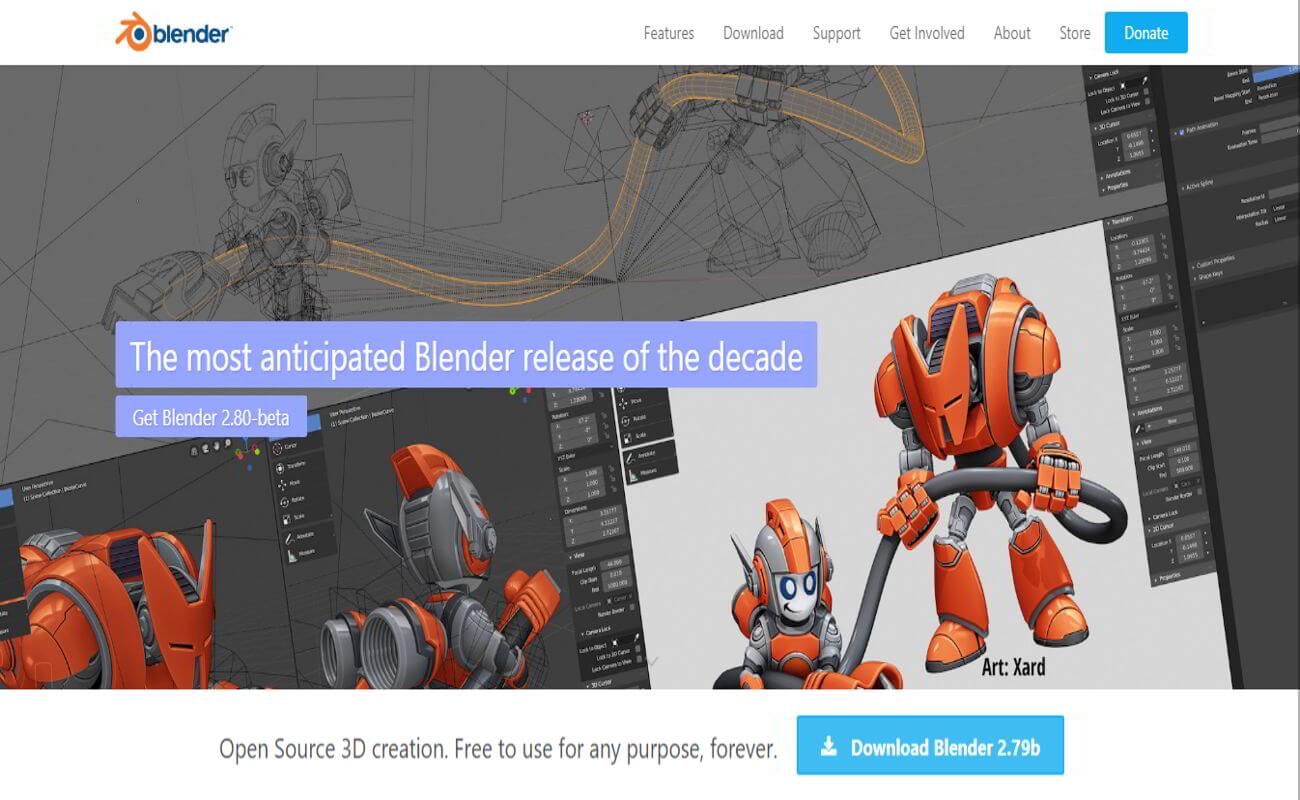A rectangular image with a landscape orientation, possibly from a video game or similar digital media, features a banner across the top left corner. The banner displays an orange circular icon with radial lines and a blue center dot, accompanied by the word "Blender" in blue text. Moving towards the banner's center, light gray text lists options: Features, Download, Support, Get Involved, About, and Store. Additionally, a blue button with white text reading "Donate" is located towards the right side of the banner.

Below the banner lies the main image. It depicts a hand-drawn character at the top, holding a hose. Another character is partially seen in the top middle area. A prominent pop-up window in the center exclaims, "The Most Anticipated Blender Release of the Decade" in white text on a purple background, with a smaller purple box below it containing the text "Get Blender 2.80-Beta" in white.

Beneath this, graphical elements showcase the main character, equipped with small jets on his back, and this character also reappears on the right side of the image.